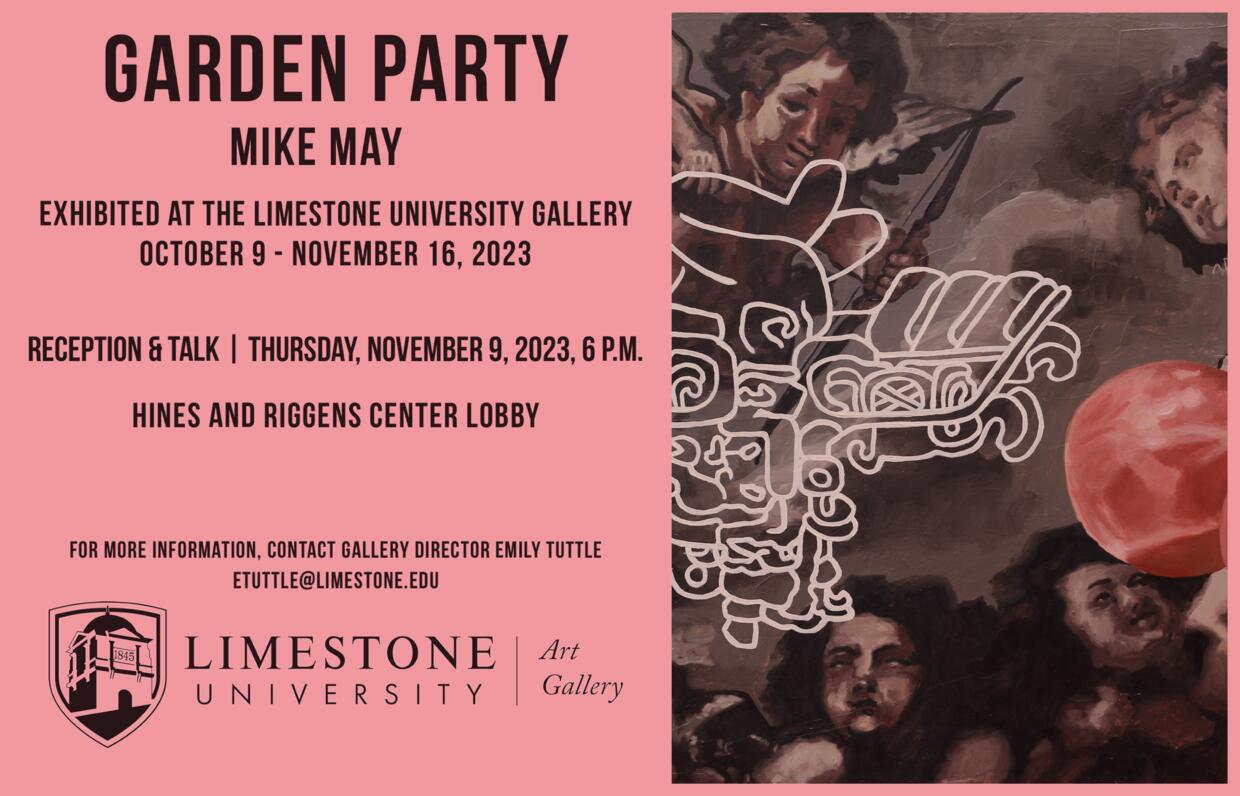The advertisement poster for the art exhibition "Garden Party" by Mike May features detailed information on the left side in dark brown text. It reads: "Garden Party, Mike May, exhibited at the Limestone University Gallery from October 9th to November 16th, 2023. Reception and talk on Thursday, November 9th, 2023, at 6 p.m. in the Hines & Riggins Center Lobby. For more information, contact gallery director Emily Toodle at etoodle@limestone.edu." At the bottom is a seal featuring a building, labeled 'Limestone University Art Gallery, 1845'. The right side of the poster displays an artistic rendering of classical cupids, depicted as naked, winged children with bows and arrows, set against a pink background with a central pink circle. The image appears to have a dingy brown hue and includes an overlay of intricate white line designs, resembling Mesoamerican art, adding a layer of complexity to the classical depiction.